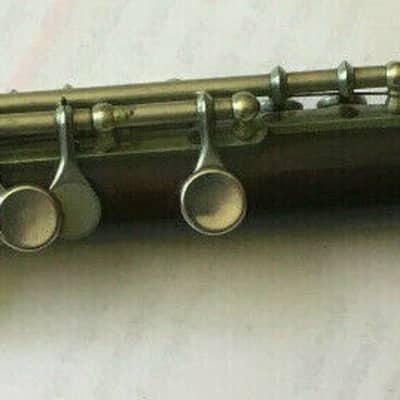The close-up image features a section of a wind musical instrument, possibly a flute, clarinet, or piccolo, laying on a white fabric surface. The photo captures three main keys or buttons made of reflective, silver-colored metal. The instrument shows signs of age, with some areas appearing slightly rusty despite its polished surface. The central key or button has a distinctive gold cylinder extending from the left to the middle of the image. Another button to the left lacks a direct finger press area and has a more silver triangular base. A circular button is mostly visible on the left of the frame. Above the central cylindrical component, there's another cylindrical alignment. The close-up nature of the photo makes it difficult to definitively identify the instrument. The image quality is poor, blurry, and marked with lines and noise, suggesting it could be a low-resolution scan with visible watermarks.